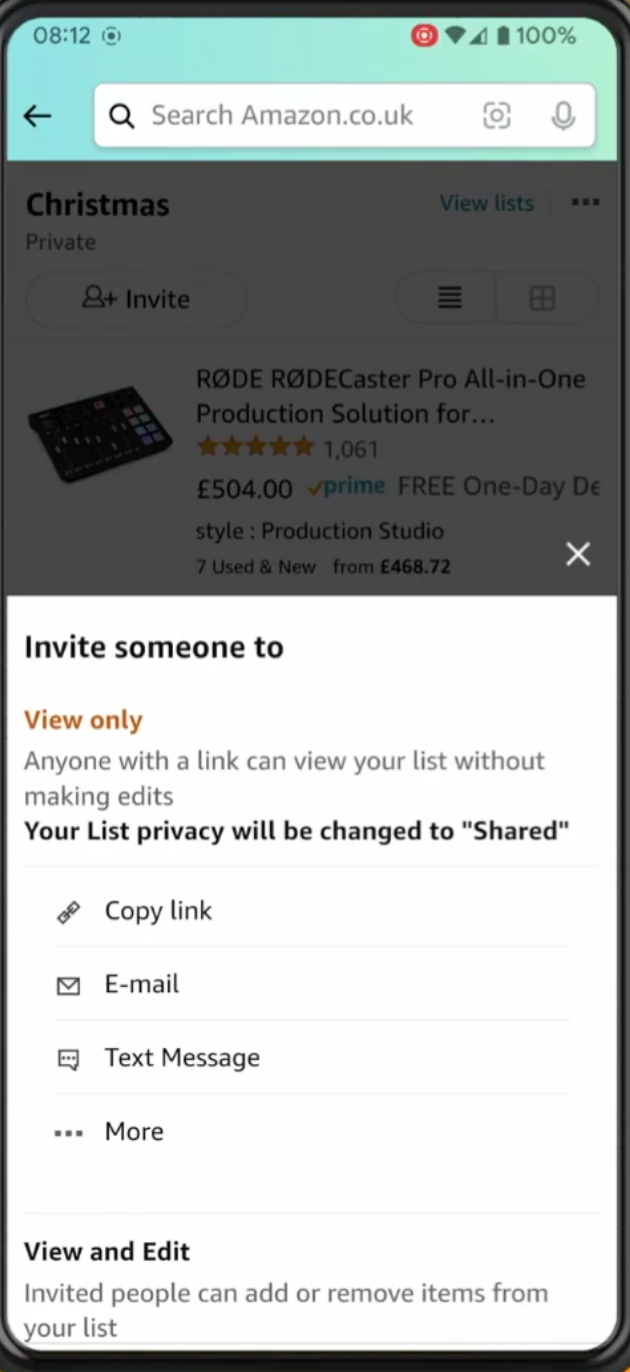Screenshot of an Amazon interface displayed on a cellphone screen. The time on the phone is 8:12, and the battery is fully charged at 100%. The top section features a blue-green search bar labeled "Search Amazon.co.uk," along with options to upload a photo or record a voice command for search, indicated by a camera and a microphone icon, respectively, along with a magnifying glass symbol.

Below the search bar, the interface slightly darkens to reveal the title "Christmas Private," indicating that the visible list is a Christmas wish list. There is a "View Lists" button prominently displayed, along with various other buttons available for adjusting the view settings.

The first item on the list is the "Rode Rodecaster Pro All-In-One Production Solution" priced at €504 and is eligible for Prime shipping. A large white box occupies the bottom half of the screen, which can be closed using an 'X' at the top-right corner. This box contains an invitation message: "Invite someone to view only. Anyone with a link can view your list without making edits. Your list privacy will be changed to shared." It provides options to copy the link, email it, send it via text message, or explore more sharing methods.

Further down, there is another option titled "View and Edit" which allows invited users the ability to add or remove items from the list, outlining various features and permissions available for managing the Amazon list.